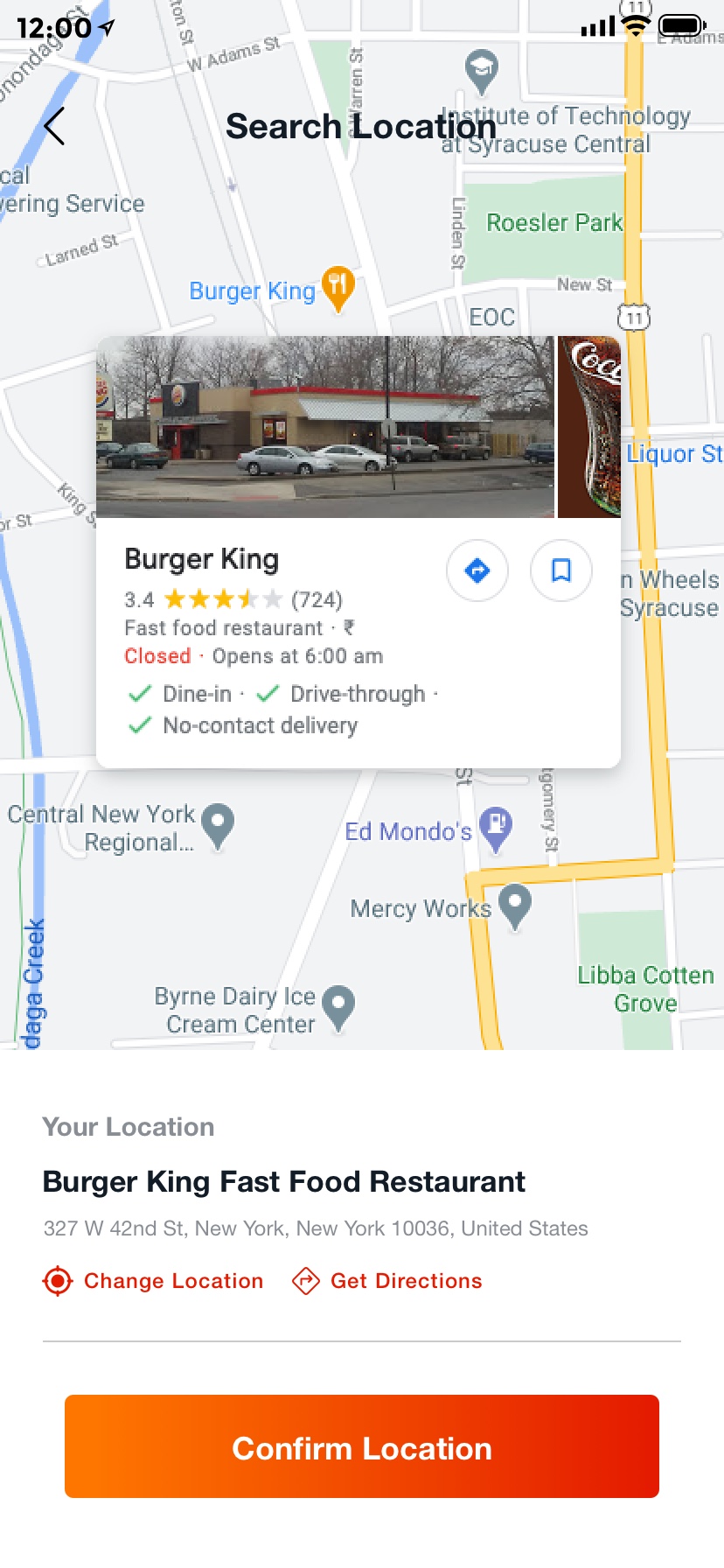This image shows a detailed screenshot of a map captured on a smartphone. The phone display indicates a full battery and a strong connection with complete signal bars. The time shown on the phone is 12:00 PM. At the top of the map, there's a search bar labeled "Search location" in black text.

The map features several pins, including orange pins indicating multiple Burger King locations and gray pins marking various other establishments in the region. A pop-up highlights one specific Burger King location, displaying an exterior image of the restaurant with cars in front. The pop-up details that the Burger King has a rating of 3.4 stars and is labeled as a fast food restaurant that is currently closed but will open at 6:00 AM. It also notes the availability of dine-in, drive-through, and no-contact delivery options.

The map itself details main thoroughfares, including Route 11 highlighted in yellow, along with other roads shown in white. Additionally, a creek appears on the map, distinguished by a blue line representing the water. Below the pop-up, the screen displays the address and name of the restaurant: "Burger King Fast Food Restaurant, 327 West 42nd Street, New York, New York, 10036, United States." Options to "Change location" and "Get directions" are shown in orange text, followed by a thin gray line. At the bottom, there is an orange box with a gradient from dark orange-red on the right to lighter orange on the left, which contains the text "Confirm location."